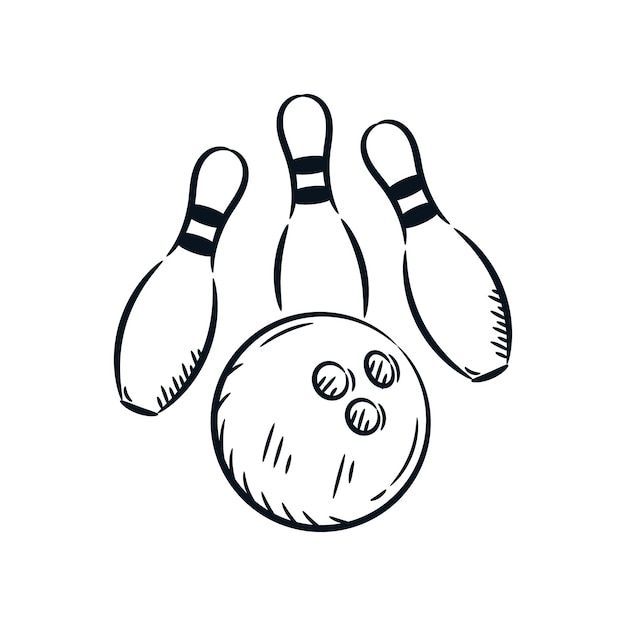This black and white illustration depicts a crudely sketched bowling scene with an emphasis on simplicity and detail. It features a bowling ball in the center foreground, detailed with three closely grouped holes, indicative of its use. Positioned behind the ball are three blue-ink drawn bowling pins, each adorned with two distinctive blue stripes near their tops. The pins appear to be tipping towards the center pin, suggesting they were recently struck by the bowling ball. Despite the lack of motion lines or any other dynamic indicators, the uneven tilt of the pins conveys a sense of recent impact, perhaps during a spare attempt. The illustration, though plain, effectively communicates the essence of the scene through its minimalist yet recognizable details.